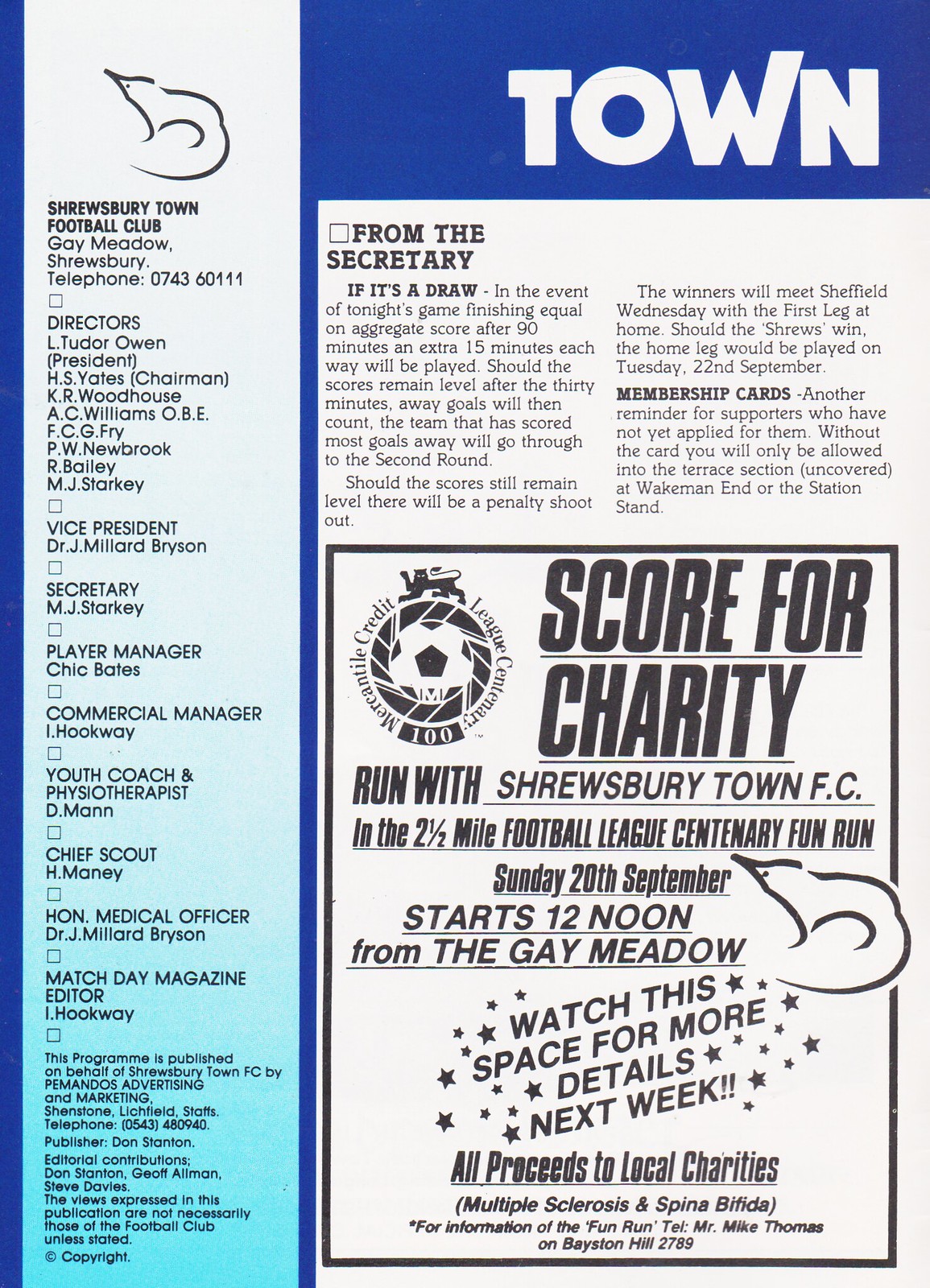This tall, rectangular advertisement for Shrewsbury Town Football Club features a striking bright blue background. On the left side, a white column fades into a light blue color and is topped with a symbol resembling a creature with a pointy nose and a tail. Beneath the symbol, "Shrewsbury Town Football Club" is printed in all capital letters, followed by several lists of names in fine print.

The right side of the image features a wide white column at the top with the bold, all-capital heading "From the Secretary." Below, the text is divided into two columns of content. Further down the right side, a prominent advertisement titled "Score for Charity" is displayed, printed in bold black letters. This section includes detailed information about the "2.5 Mile Football League Centenary Fun Run" happening on Sunday, September 20th, starting at noon from the Gay Meadow, encouraging participation and noting that all proceeds will support local charities.